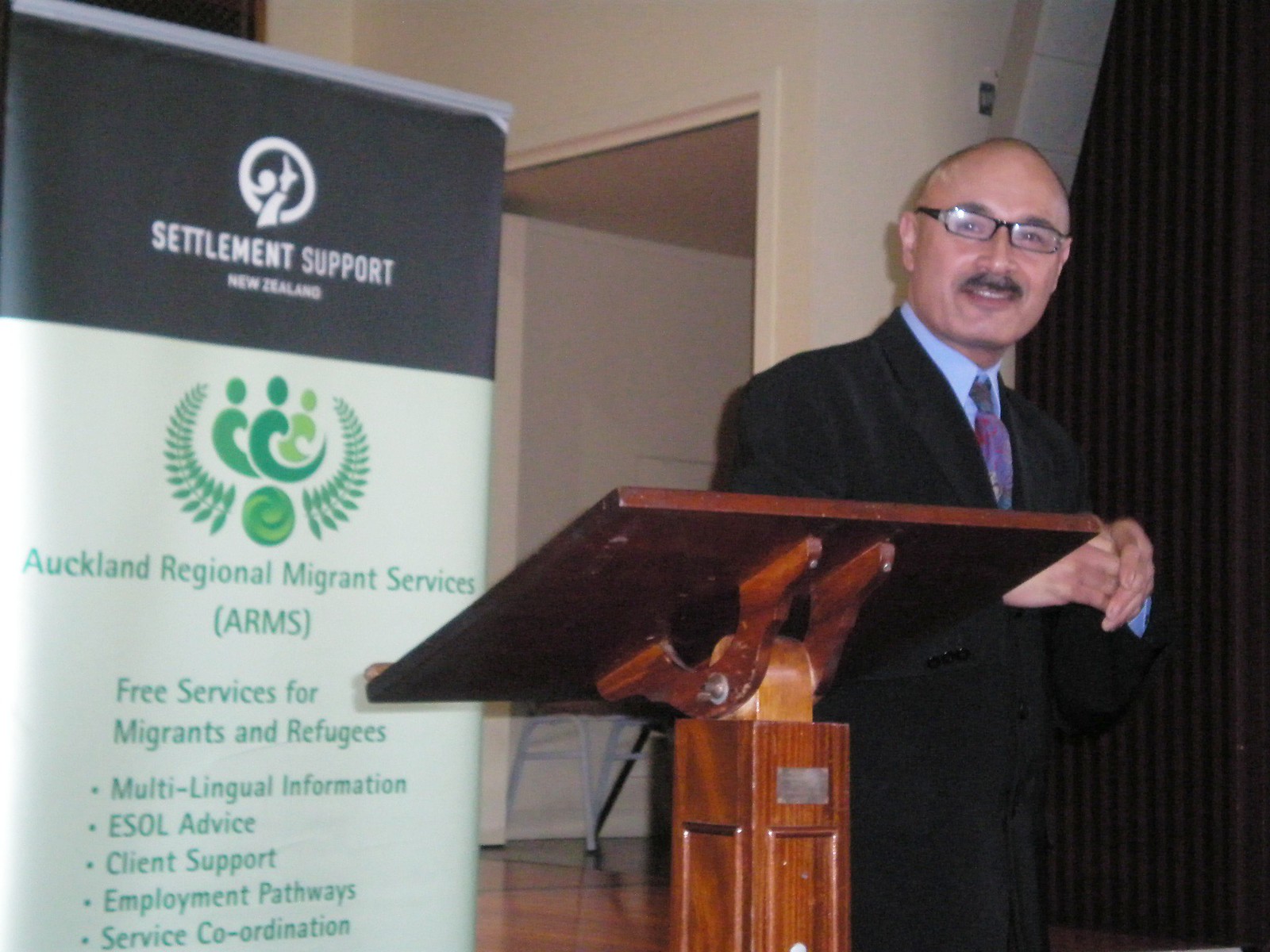A man with a black mustache and thin black glasses, standing to the right of a wooden podium, smiles warmly at the camera, with his hands clasped together in front of his chest. His short hair, showing a bit of gray at the sides and light stubble on top, complements his black suit, blue shirt, and multicolored tie composed of purple, pink, and black hues. Behind him, a doorway opens into a hallway, while to the right, a black curtain or closed door with vertical lines is visible. The podium, centered in the scene, features a sturdy 4x4 post and adjustable components secured by wingnuts. To the left of the podium, a large banner reads "Settlement Support New Zealand" in white text on a black background, followed by "Auckland Regional Migrant Services, a.k.a. ARMS, Free Services for Migrants and Refugees, Multilingual Information, ESOL Advice, Client Support, Employment Pathways, and Service Coordination" in green text on a white background. The banner, exuding a sense of community and support, signifies the event's focus on aiding migrants and refugees.